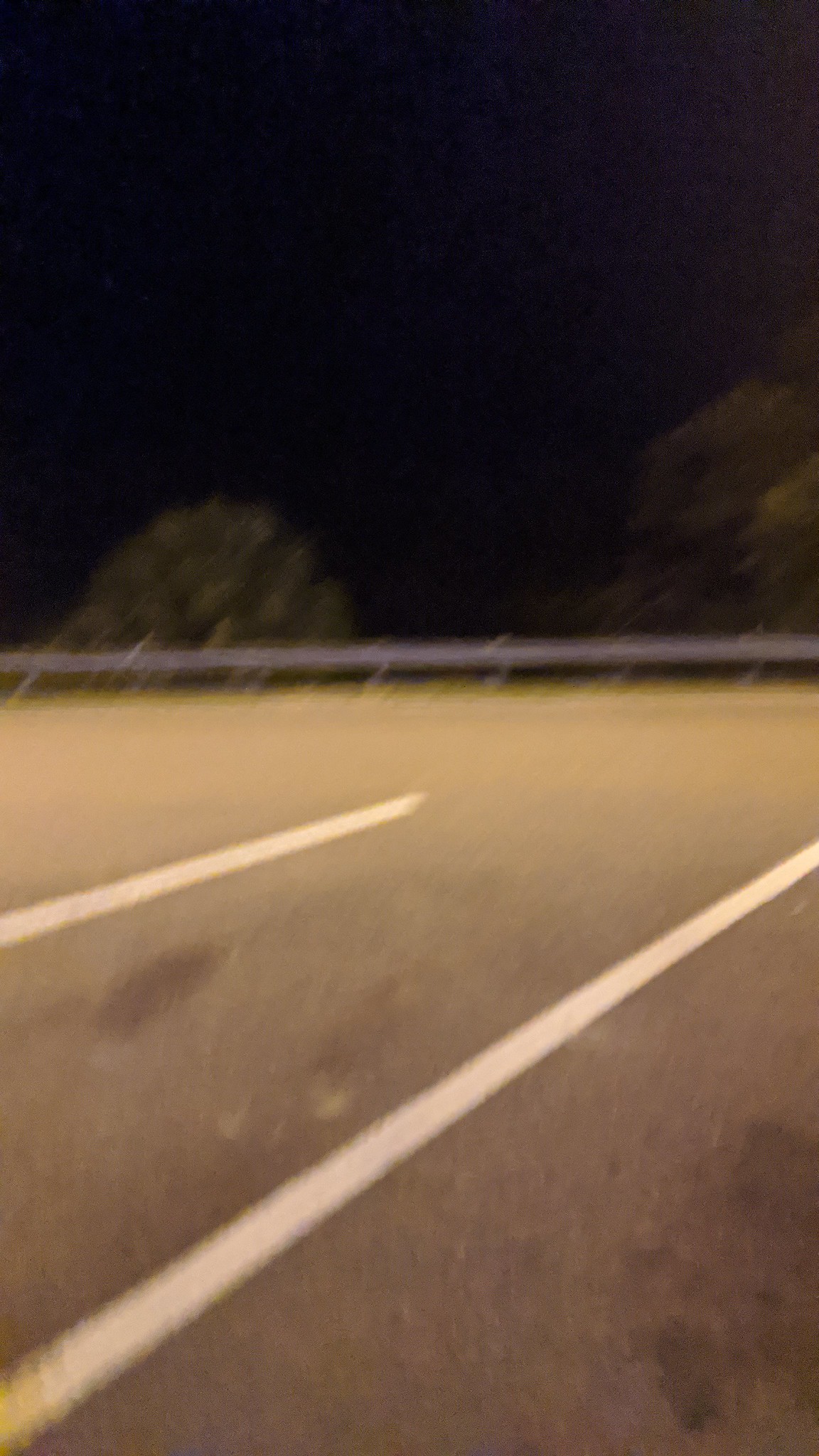Despite the blurry, low-resolution quality of the image, it clearly depicts an outdoor scene at night. The sky is pitch black, emphasizing the nighttime setting. Below, the ground appears gray with two distinct white lines marking its surface. A gray rail stretches horizontally from left to right in the midground, providing a sense of structure. In the background, a row of green trees is visible behind the rail, adding a natural element to the scene.